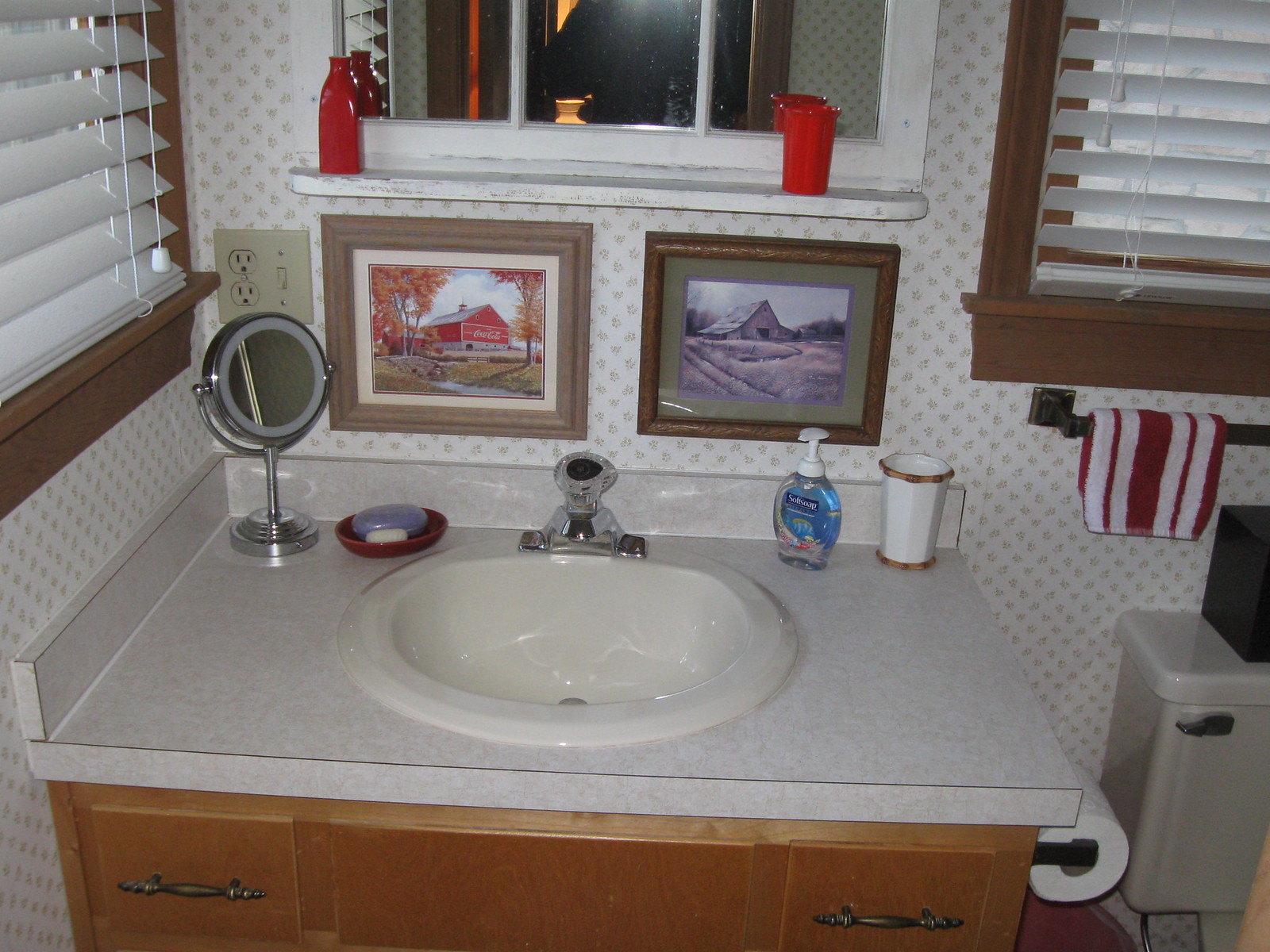This image depicts a cozy corner bathroom with meticulous details. On the left side, there are two windows. The window in the foreground has a brown frame adorned with white blinds. In the center of the image, the base of the basin is visible. It features a brown cupboard with a white countertop, which boasts a grey-white marble texture. A sink is embedded in the countertop.

Additionally, there is a small, portable circular mirror with a silver frame placed on the basin counter. Behind this mirror, there is a plug socket with two plug openings. The wallpaper of the bathroom is white with a subtle dotted design.

Above the basin, a large mirror with a white frame is mounted, flanked by two red decorative accents on each side. Below this main mirror, there are two picture frames. The left frame is greyish and contains an image of a red farmhouse surrounded by red trees. The right frame is brown and features a picture of a house situated in the woods.

On the basin countertop, there are several items, including a soap bar holder that contains one purple and one white soap bar. Next to it is a colorless hand wash bottle with a blue label and a white pump lid, accompanied by a white cup with decorative designs at the top and bottom.

To the right of the basin, there is another window identical to the one on the left. Below this window sits a tissue holder with a roll of tissue and a small towel rail displaying a red and white towel. In the bottom right corner, a portion of the toilet is visible, featuring a black cover.